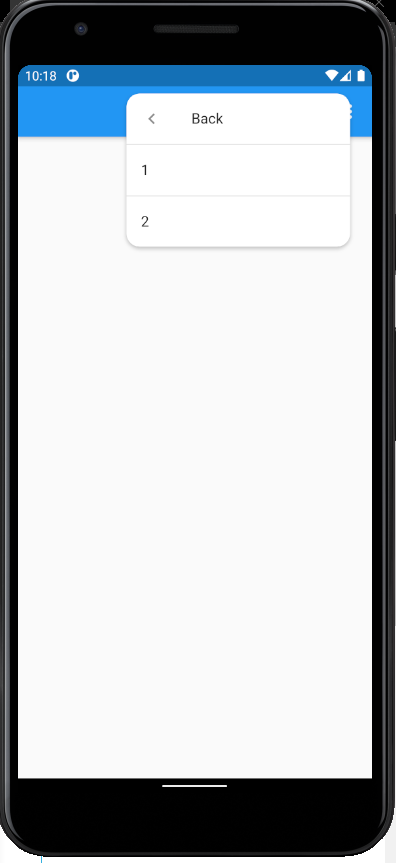The image showcases a smartphone screen with visible rounded borders. The screen is primarily white, with significant empty space and two prominent horizontal blue bars. The topmost, a navy blue bar, displays the time "10:18" alongside a circular icon whose purpose isn't clear. Adjacent to the time display, toward the right side, there is an icon resembling a baseball field diamond, indicating zero reception bars, followed by a triangle symbol representing battery life. Below this is a thicker blue bar, and within this bar is a window with rounded corners, displaying three rows of content. The first row contains a back arrow symbol, commonly used to navigate to the previous screen. The following two rows contain the numbers "1" and "2" respectively. The overall design is minimalist, emphasizing the ample white space on the smartphone screen.